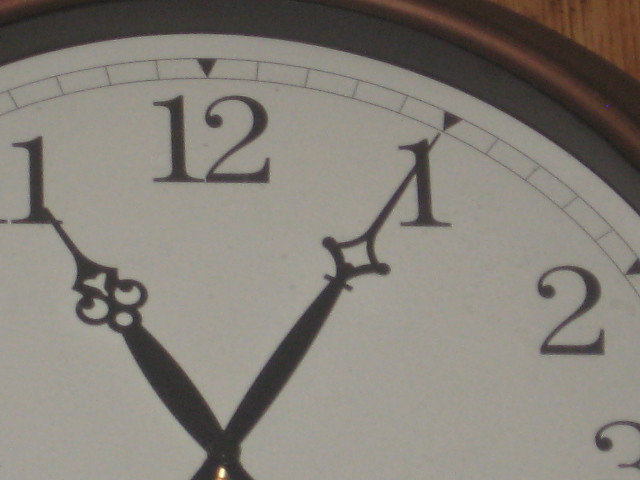The image is a close-up, color photograph of the upper right portion of an analog clock face. The visible section of the clock shows the numbers 11, 12, 1, 2, and part of the 3. Notably, the number 1 from the 11 is also in view through the upper left segment of the image. The clock's design features a dark brown, circular bezel, which has a metallic, almost bronze-colored raised portion separating inner and outer edges of the frame. The face itself is white with big black numbers and a subtle pattern of black squares, each with black arrows pointing inward toward the center of the clock. The clock hands are black and pointed: the minute hand is pointing at the 1, indicating five minutes past 11, while the hour hand points directly at the 11. Behind the clock, a panel of vertically-grained mahogany wood with dark lines is visible, though it is unclear whether the clock is mounted on a wall or lying face-up on a table. The center of the clock, where the hands are mounted, is a gold color, and the structure is accentuated by a small, brown ball-like detail in the top right corner.